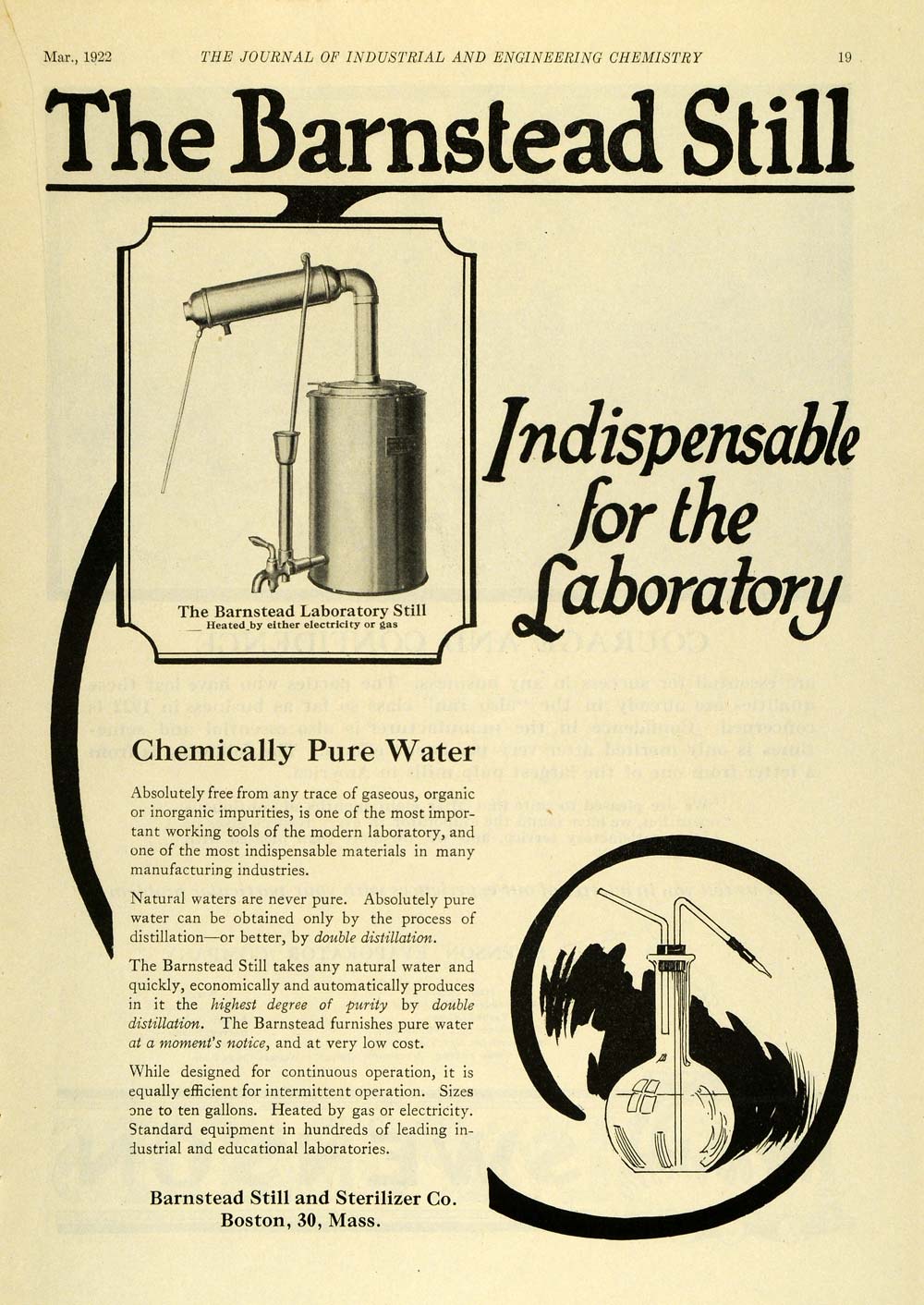The image is a faded light yellow page taken from the Journal of Industrial and Engineering Chemistry, dated March 1922, labeled as page 19. At the top, written in bold, black letters, is the article title "The Barnstead Still," underlined with a black line that extends and wraps around to the left. The central illustration features a detailed depiction of the Barnstead still: a silver cylinder with a pipe extending from the top that curves to the left and enlarges, ending in a nozzle-like structure, and a long string descending towards the bottom left. This main image is set within a square with curved cut-outs at the corners.

Below the main image are four paragraphs of text extolling the virtues of the Barnstead still, describing it as indispensable for the laboratory and capable of producing chemically pure water free of all impurities. The text further elaborates that the still provides purified water quickly, economically, and automatically, making it a vital tool for both laboratories and manufacturing industries.

On the right side of the page is additional text emphasizing the still's necessity for laboratory work. At the very bottom right, there is another illustration of a round-bottom beaker with two straws – one straw going up to the left and another bending back down to the right, set against a background with black paint etchings. The bottom of the page is signed off with "Barnstead Still and Sterilizer Company, Boston, 30 Mass."